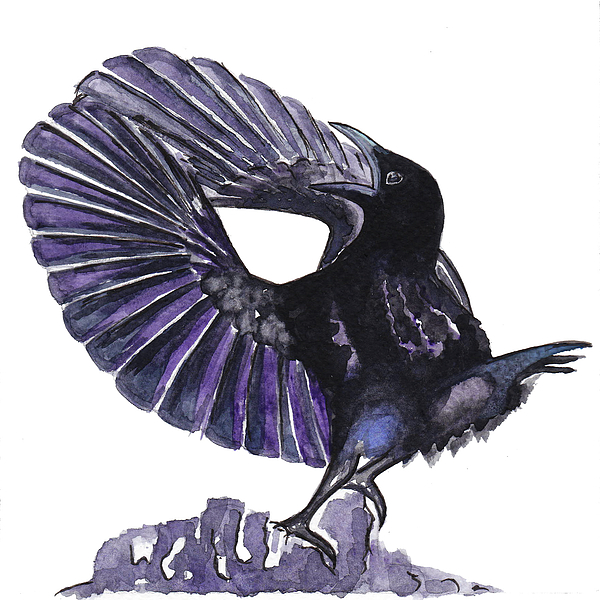This vertical artwork, which has no external border and appears to be a watercolor painting or an animated picture, features a dark blue bird, likely a raven, standing on gray or purple rocks against a completely white background. The bird, facing to the left with its mouth slightly open, showcases a detailed design with dark blue tail feathers that transition to a lighter blue at the end. Its beak is gray, and one visible eye is black outlined in white. The bird’s wings, spread out in a circular pattern, connect and form a ring-like structure in front of its beak. These wings are primarily purple, with the right wing displaying a lighter shade. The wings also feature purple lines that intricately represent feathers, adding to the abstract and detailed nature of the artwork.